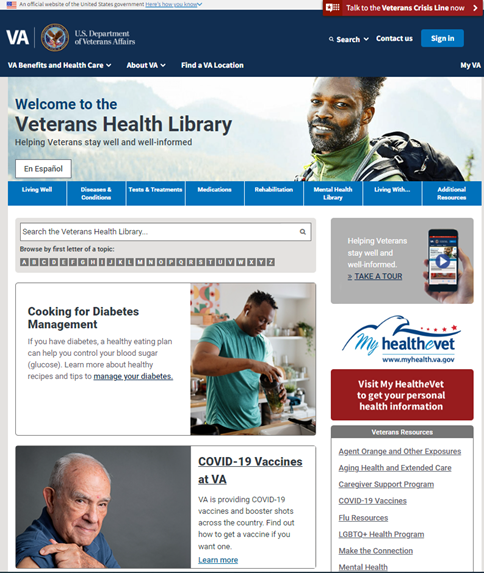The image showcases a screenshot of a U.S. Department of Veterans Affairs website, designed to provide information and resources to veterans. 

At the top, there's a small beige banner featuring the American flag, with the text, "An official website of the United States government. Here's how you know," linked as a blue hyperlink. On the right side, a prominent red banner reads, "Talk to the Veterans Crisis Line now," with an arrow pointing to the right for immediate assistance.

Beneath these banners, a navy blue banner displays "VA | U.S. Department of Veterans Affairs" in white text. This is followed by navigation options:
- "VA Benefits and Healthcare" with a drop-down menu.
- "About VA" with a drop-down menu.
- "Find a VA Location."
- Another drop-down menu for "Search" with "Contact Us."
- "Sign In," and "My VA."

The main content area features a background image of a person set against a mountainous landscape under a clear sky. It is accompanied by the message, "Welcome to Veterans Health Library. Helping veterans stay well informed," with an option to switch to Spanish ("Español").

A blue banner lists categories such as:
- Living Well
- Diseases and Conditions
- Tests and Treatments
- Medications
- Rehabilitation
- Mental Health Library
- Living with ...
- Additional Resources

Below these categories, a search bar reads "Search the Veterans Health Library," followed by featured topics like "Cooking for Diabetes Management" and "COVID-19 Vaccines at VA."